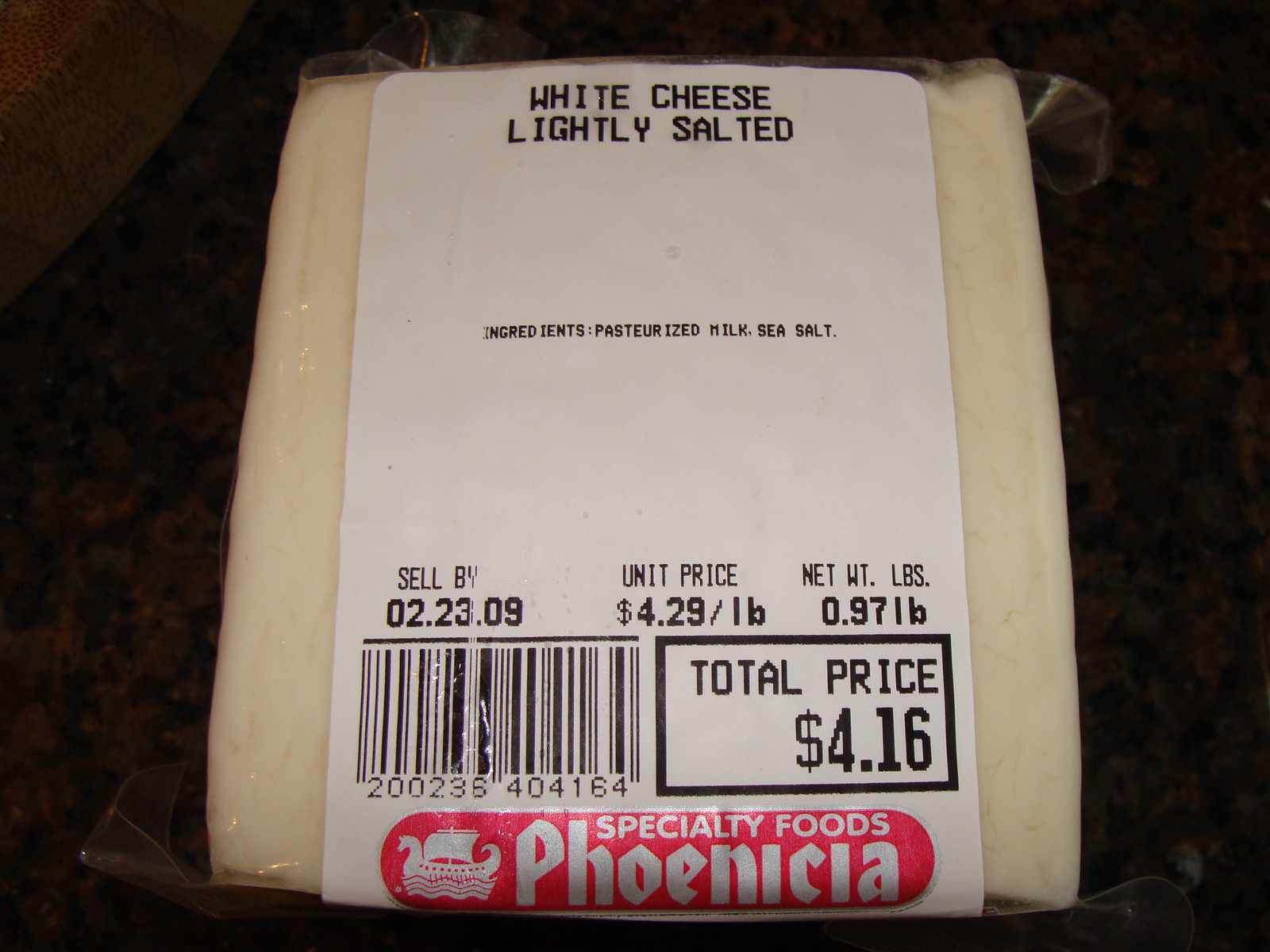The image captures a close-up of a horizontally oriented piece of cheese, packaged in clear plastic with a white label. The cheese, described as "white cheese lightly salted" in bold, black capital letters, has an eggshell white to yellowish color. The label provides detailed information: ingredients include pasteurized milk and sea salt, while the net weight is 0.97 pounds. The total price is $4.16, with a unit price of $4.29 per pound. A sell-by date of February 23, 2009, is printed above a black barcode. The packaging also features a red oval label at the bottom with the text 'Specialty Foods Phoenicia' and an illustration of a Phoenician boat. The background of the image consists of a zoomed-in marble surface in shades of brown, black, and a bit of white, though it's unclear if the surface is a counter or a table due to the tight crop of the photo.